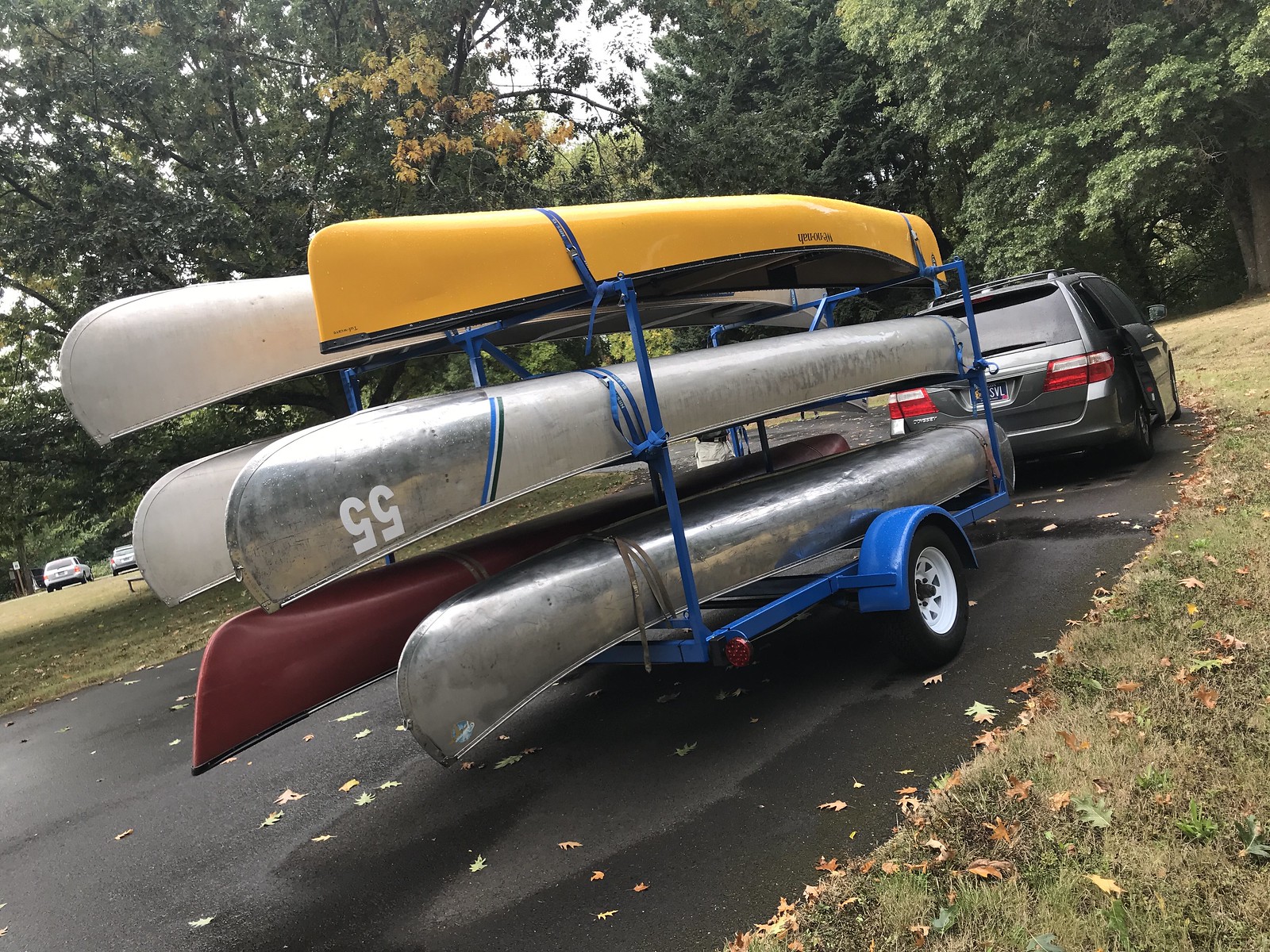The photograph depicts a gray minivan, with its back door slid open, stationary in a parking area surrounded by grass. The minivan is connected to a blue trailer loaded with six canoes of varying colors and sizes. The canoes are arranged in two rows of three; the back row contains two white canoes and a maroon one on the bottom, while the front row includes a smaller yellow canoe on top, a silver canoe with the number '55' in white lettering in the middle, and another silver canoe at the bottom. The canoes are positioned on a small asphalt strip amidst a park-like setting. It's autumn, evident from the leaves turning color in the trees and some fallen leaves scattered on the ground, with a hint of moisture indicating recent rain. In the distance, the image captures a couple of other cars in a concrete parking area, bordered by a grouping of trees with a small clearing revealing the sky.